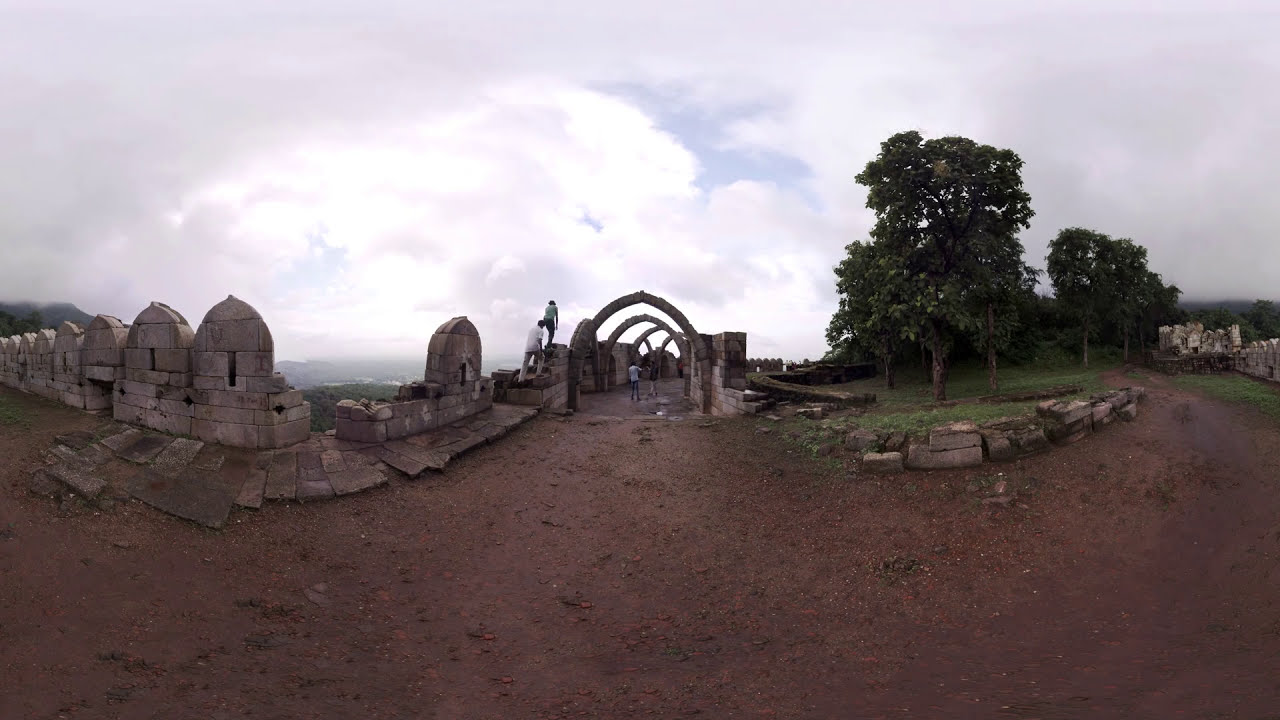This panoramic photograph, likely created by stitching together multiple images, depicts an ancient archaeological site, possibly an old church or castle complex. The scene is captured outdoors during the daytime, under a sky filled with clouds that darken towards the corners, with glimpses of blue peeking through the brighter center. The foreground is dominated by a dark brown, almost reddish dirt pathway, and scattered patches of grass and a small grove of trees.

Central to the image is a series of stone ruins featuring prominently arched remnants, with no remaining roof, suggestive of a once-grand structure now in decay. To the left, a stone wall built of large, gray bricks overlooks what might be a cliffside, with each brick topped in a smooth, curved arch. In the middle distance, you can discern two people climbing on the ruins and another pair, much smaller due to the photo's scale and distance, standing beneath one of the central archways. To the right, additional ancient stone walls complete the scene, adding to the sense of a sprawling, historically rich site. The photo exhibits a slight warping effect, characteristic of a 360-degree camera, which curves the edges of the image into an extreme curvature, lending a unique, almost surreal quality to the overall composition.